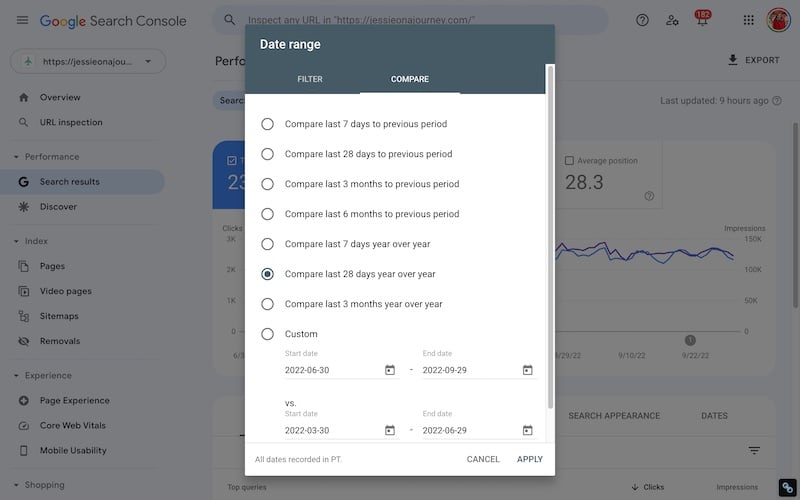The image depicts a detailed view of the Google Search Console interface. On the left-hand side of the screen, the main navigation menu is visible, allowing users to access various tools and reports. Dominating the right-hand side is the performance dashboard, providing insights into website metrics.

Centrally featured in the image is a prominent rectangular modal focused on date range selection, offering robust comparative analysis options. This modal includes two primary functions: "Filter" and "Compare," the latter of which is highlighted to indicate its active selection.

Within the "Compare" section, multiple pre-set comparison options are presented:
- Compare the last 7 days to the previous period
- Compare the last 28 days to the previous period
- Compare the last 3 months to the previous period
- Compare the last 6 months to the previous period
- Compare the last 7 days year over year
- Compare the last 28 days year over year
- Compare the last 3 months year over year

Additionally, users are provided with the flexibility to select custom date ranges. This feature includes two side-by-side fields, each with a start date picker and an end date picker, allowing for comprehensive temporal analysis.

Beneath these options lies a horizontal divider bar. On the left-hand side of this modal, it notes that all dates are recorded in Pacific Time (PT). Towards the bottom right corner of the modal, two buttons are present: "Cancel" on the far left and "Apply" immediately to its right, assisting users in finalizing their selections.

A vertical scroll bar is also visible on the right side of the screen, indicating that more options or data might be accessible through scrolling. The "Compare" feature is prominently highlighted, ensuring users can easily identify and utilize this function for their analysis.